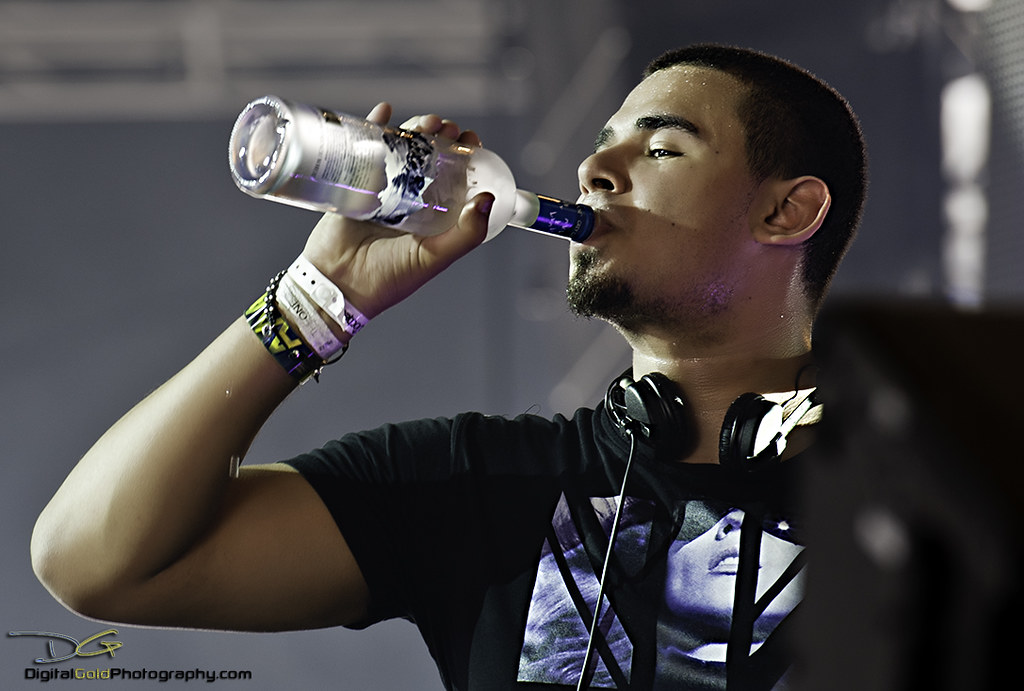The photograph captures a young man drinking straight from a tequila bottle, visible only from the chest upwards with his left side out of frame. Positioned towards the center, he wears a short-sleeved black graphic t-shirt featuring the lower half of a woman's face with an ocean wave background. Over his neck sits a pair of over-the-ear headphones, a wire hanging down. He has short black hair and a goatee, suggesting a youthful appearance. A black computer monitor faces him from the right side of the image, while the background remains blurred. In the bottom left corner, a watermark in silver and gold reads "DG" with "digitalgoldphotography.com" below in smaller text.